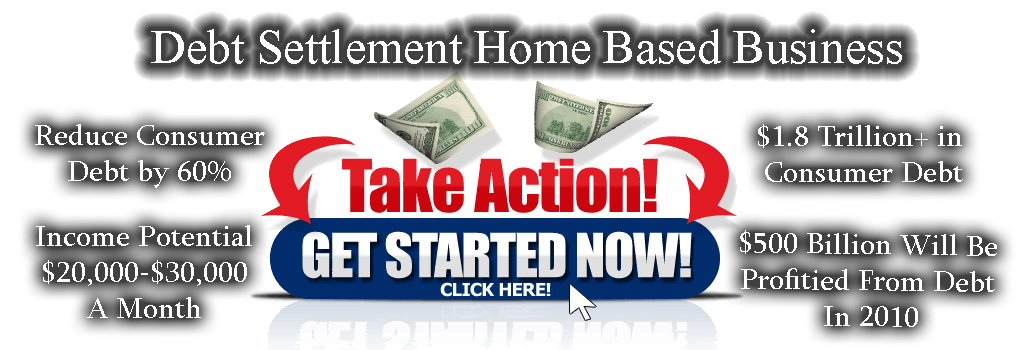This vibrant advertisement, likely sourced from a website, features a predominant white background with gray and white text at the top reading "Debt Settlement Home-Based Business." The text is accentuated by a shadow effect, enhancing its visibility. Centrally positioned, two folded $100 bills catch the eye above the bold red phrase "Take Action!" Two red arrows direct attention downward to a blue, pill-shaped button that says "Get Started Now - Click Here," accompanied by a mouse cursor icon. On the left, the ad highlights benefits with "Reduce Consumer Debt by 60%" and notes the impressive "Income Potential: $20,000 to $30,000 a Month." On the right, it underscores the substantial economic impact with "1.8 Trillion Plus in Consumer Debt" and "500 Billion Dollars Will Be Profited From Debt in 2010." This comprehensive graphic emphasizes lucrative opportunities within the debt settlement industry.